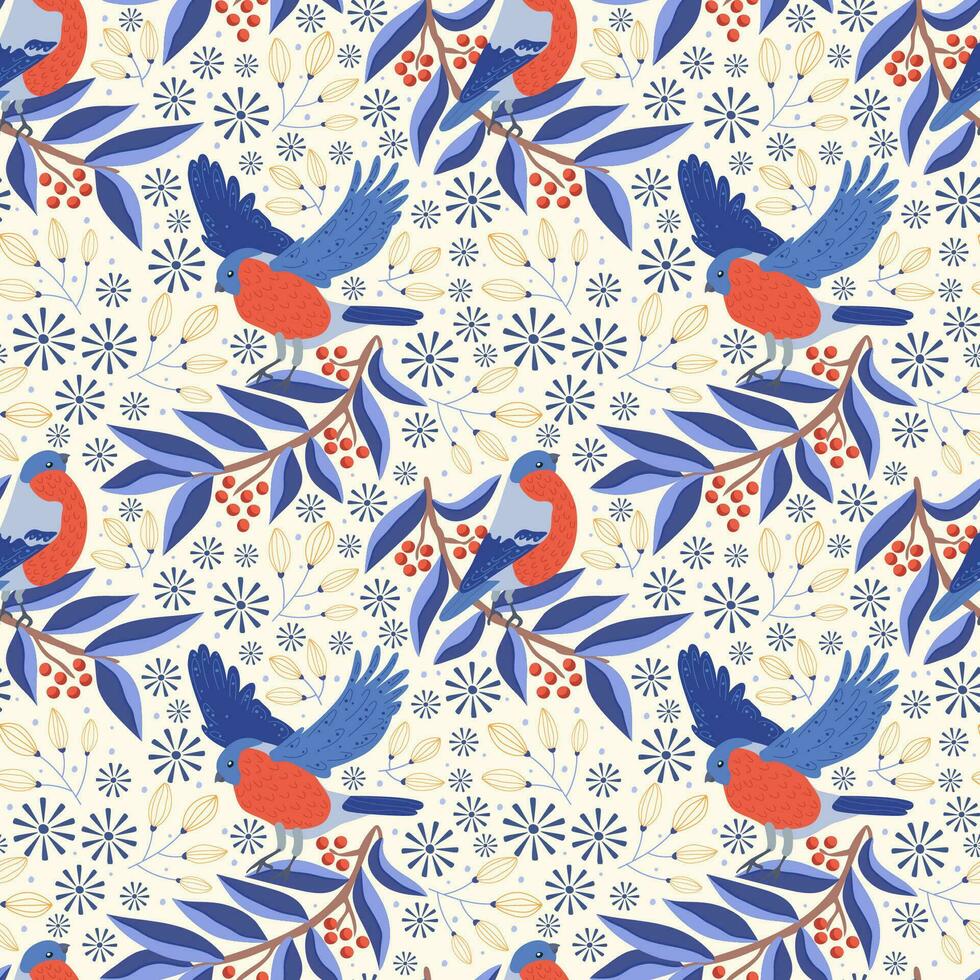The image features a detailed, repeating pattern that could be used as wallpaper, a textile, or even wrapping paper. The background is primarily cream or white. The central elements of the design are blue birds with light blue and dark blue wingtips, orange breasts, and grayish-black beaks and eyes. These birds are shown in different positions: some facing left with their wings extended, and others facing right while perched on branches or leaves. 

The branches themselves are brown with blue and white leaves, some of which are dual-toned with light and dark blue. Interspersed among the branches are red berries and various floral elements, including unopened goldish blossoms, white buds, and starburst-shaped blue flowers. These floral and botanical details add splashes of white, red, blue, and a touch of yellow to the overall pattern.

The design showcases a seamless repetition of these elements, with patterns of birds, branches, and flowers appearing in an orderly sequence across the surface. This comprehensive combination of colors and intricate details creates an elegant and harmonious visual.